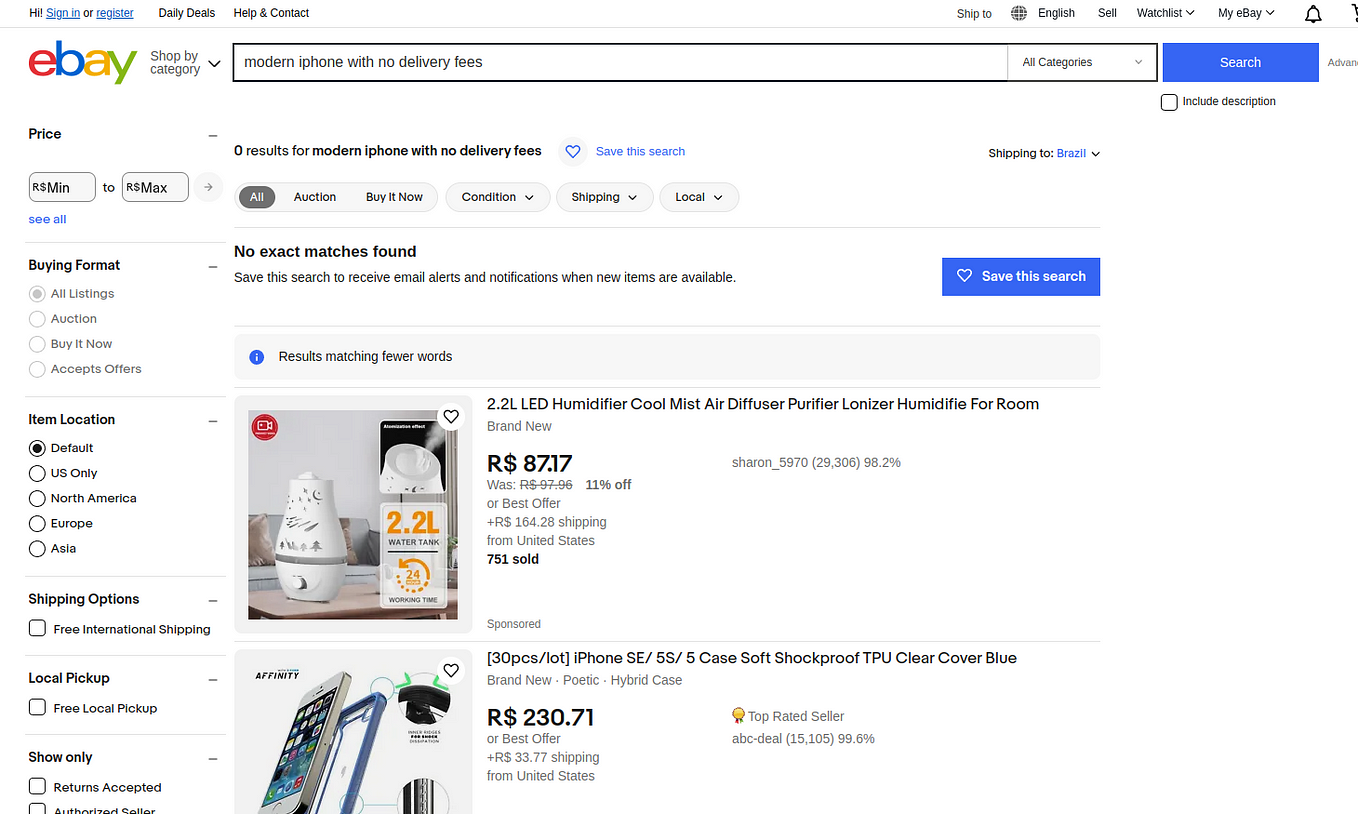This detailed caption highlights various elements visible in the image, which is a screenshot of an e-commerce website, likely eBay:

---

The screenshot showcases a user interface from an e-commerce website, evidently, eBay. Key elements visible in the header include links for "Hi, Sign In," "Register," "Daily Deals," "Help & Contact," "Worship 2," "English," "Sell," and "Watchlist," as well as icons for "My eBay." The eBay logo is prominently displayed beside a navigation option labeled "Shop by Category."

A modern iPhone advertisement highlights "No Delivery Fees," and categories such as "All Categories," "Square," "Search," "Advanced," and "Include Description" are presented. Below, various filter options like "Price," "Min to Max," "Point Format," "All Listings," "Auction," "Buy Now," and "Microsoft Advocation" are shown.

Further filtering options include "Default," "US Only," "North America," "Europe," "Asia," and "International Shipping." The interface also displays options for "Free Local Pickup," "Transcriptor," "Seller," and indicates "Zero Results for Modern iPhone with No Delivery Fees." 

Sections for "Accessories," "Shipping to Brazil," "All Auction," and "Buy Now" are also visible. Conditions like "Shipping Local," notes mentioning "Matching is Found," with options to "Save the Search," and receive "Receipt," "Email," "Alerts," and "Notifications" when new ads are posted, are present as well.

Highlighted is an advertisement for an LED Humidifier, described as a "2.2 Liters, Cold Mesh, Turn Off, Pre-Fire, Ionizer, Humidifier for Room," priced at "87.17 Rubles." 

Additional items featured include a "White Shirt," notes on "30 Pieces," a "White Phone," and references to "Etsy," "Slash 5, Slash 5K," "Soft," "Chakra," "TPU Clear Cover Blue," listed as "Brand New," from "Bode Kybergate," with a price of "230.71" and a "Best Offer" option.